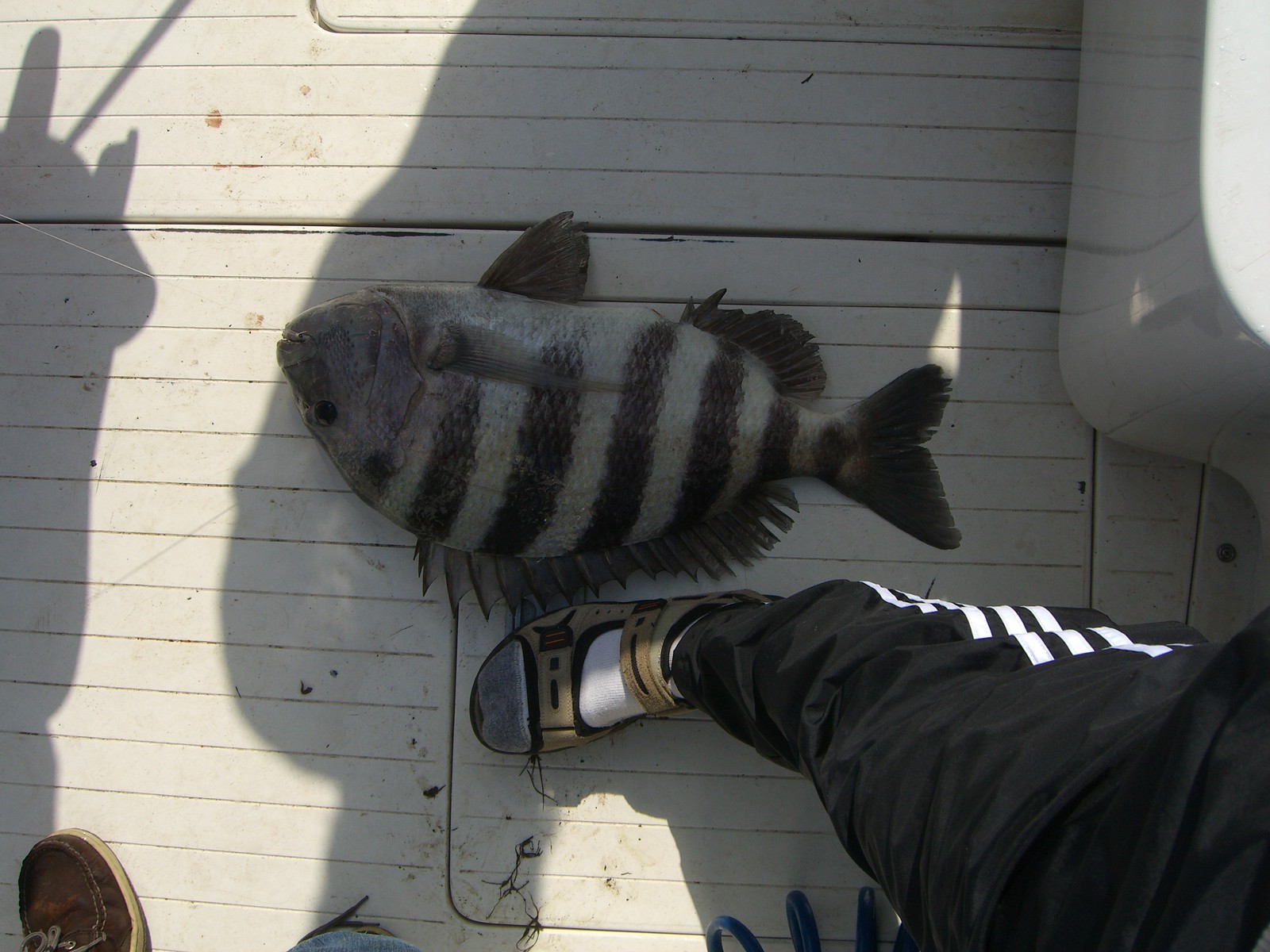The image captures the deck of a boat, featuring a scene from a fishing expedition. Central to the composition is a large, stout gray fish with darker gray and black stripes, lying upside down relative to the photo's orientation. The fish is notably wide and measures about two to three times the length and twice the width of the visible person’s foot. This foot, encased in a white sock and beige sandal, belongs to someone wearing black sweatpants with white stripes. Adjacent to the fish, there's another foot clad in a brown shoe. Adding depth to the scene, the shadow of a person holding a fishing pole stretches across the white, beige-striped deck, grounding the image in the context of a fishing adventure.